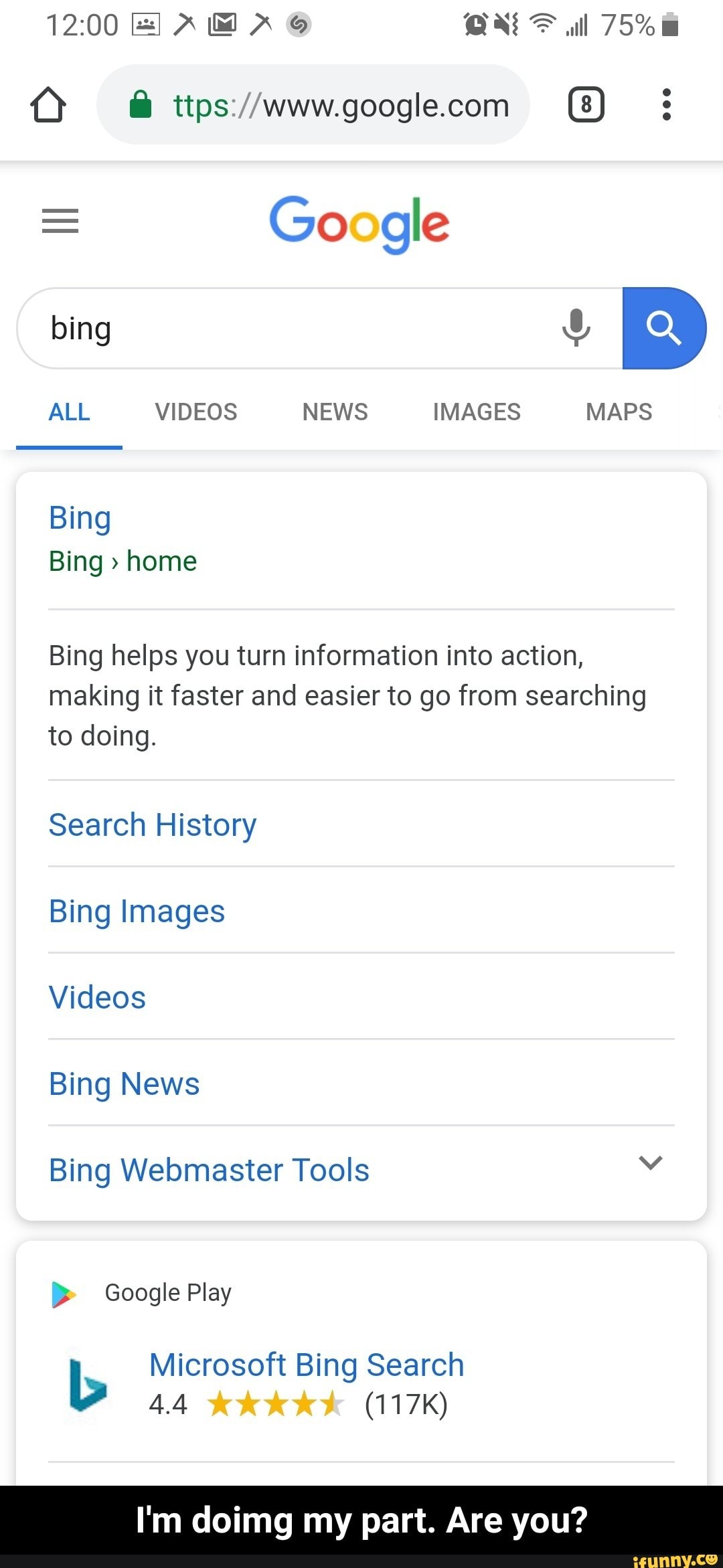A detailed and cleaned-up caption for the described smartphone screenshot could be:

---

A screenshot of a smartphone displaying a web browser at 12:00 PM. The status bar shows icons for groups (represented by a pickaxe), email, a second pickaxe, an icon resembling the number '69' within a gray circle, a clock, a muted sound icon, Wi-Fi, and a battery at 75%. The browser's interface includes a home icon and a search box displaying “www.google.com,” with eight tabs open and a menu represented by three vertical dots. Below is a hamburger menu and the Google logo.

The main search bar below the logo contains the word "Bing," accompanied by a microphone icon and a magnifying glass icon. The navigation tabs beneath the search bar include options for 'All' (currently selected), Videos, News, Images, and Maps.

Further down, the content section starts with the term "Bing" followed by a forward arrow and the word "Home." Beneath a light gray line, there is a description: "Bing helps you turn information into action, making it faster and easier to go from searching to doing." This is followed by segments titled 'Search history' in blue, 'Bing images' in blue, 'Videos' in blue, 'Bing news,' 'Bing webmaster tools' with a drop-down arrow, each separated by thin gray lines.

At the bottom of the screen, there is a Google Play logo, followed by a Microsoft Bing logo along with "Microsoft Bing search, rated 4.4 stars from 117,000 votes." The final visible line reads "I'm doing my part, are you?"

---

This caption provides a structured and detailed description of the smartphone screenshot as described.